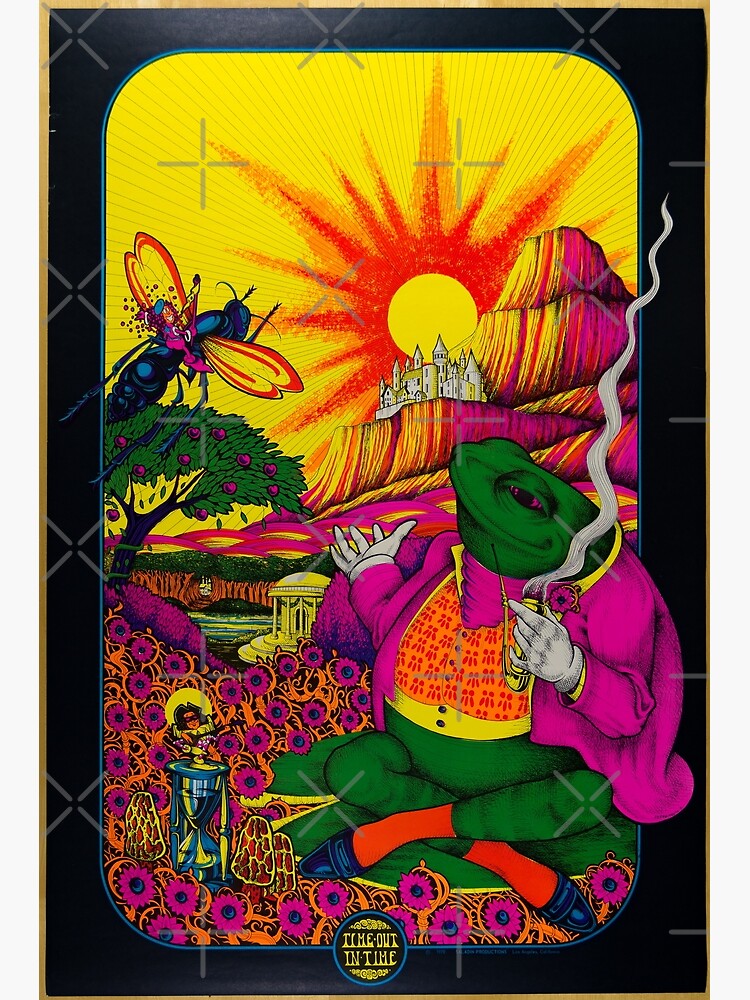This artist’s rendering has the intricate detail of a playing card or a vivid poster, perfect for framing and hanging. The image is set within a goldish-brown and black border, giving it an ornate and finished look. At the center of this vertical artwork sits a large, anthropomorphic green frog on the right, positioned like a person. The frog is immaculately dressed in a bright purple jacket, a purple scarf tied around its neck, and an eye-catching orange vest trimmed with yellow, adorned with dark buttons. Completing its ensemble are orange socks and dark dress shoes, with a decorative pipe in its left hand, gently emitting smoke.

The frog is nestled among vibrant flowers and whimsical mushrooms, creating a lush foreground filled with rich details. An hourglass with a small person peeking out from the top adds to the scene's whimsical charm. Adjacent to this is a gazebo, painted in golden hues, surrounded by more trees that extend into the distance. Above this dreamy landscape, the sky is a mixture of psychedelic colors with a radiant yellow sun that has red and orange rays extending outward. Pink fruits adorn a tree to the left, and a colossal dragonfly with a smiling, pink-clad figure riding atop bursts into the scene, adding a fantastical twist.

Background elements include pink, yellow, and orange mountains, a light gray castle situated below the beaming sun, and additional trees that weave through the upper backdrop. Every inch of this piece is filled with brilliant colors and meticulous detail, making it a mesmerizing visual feast.